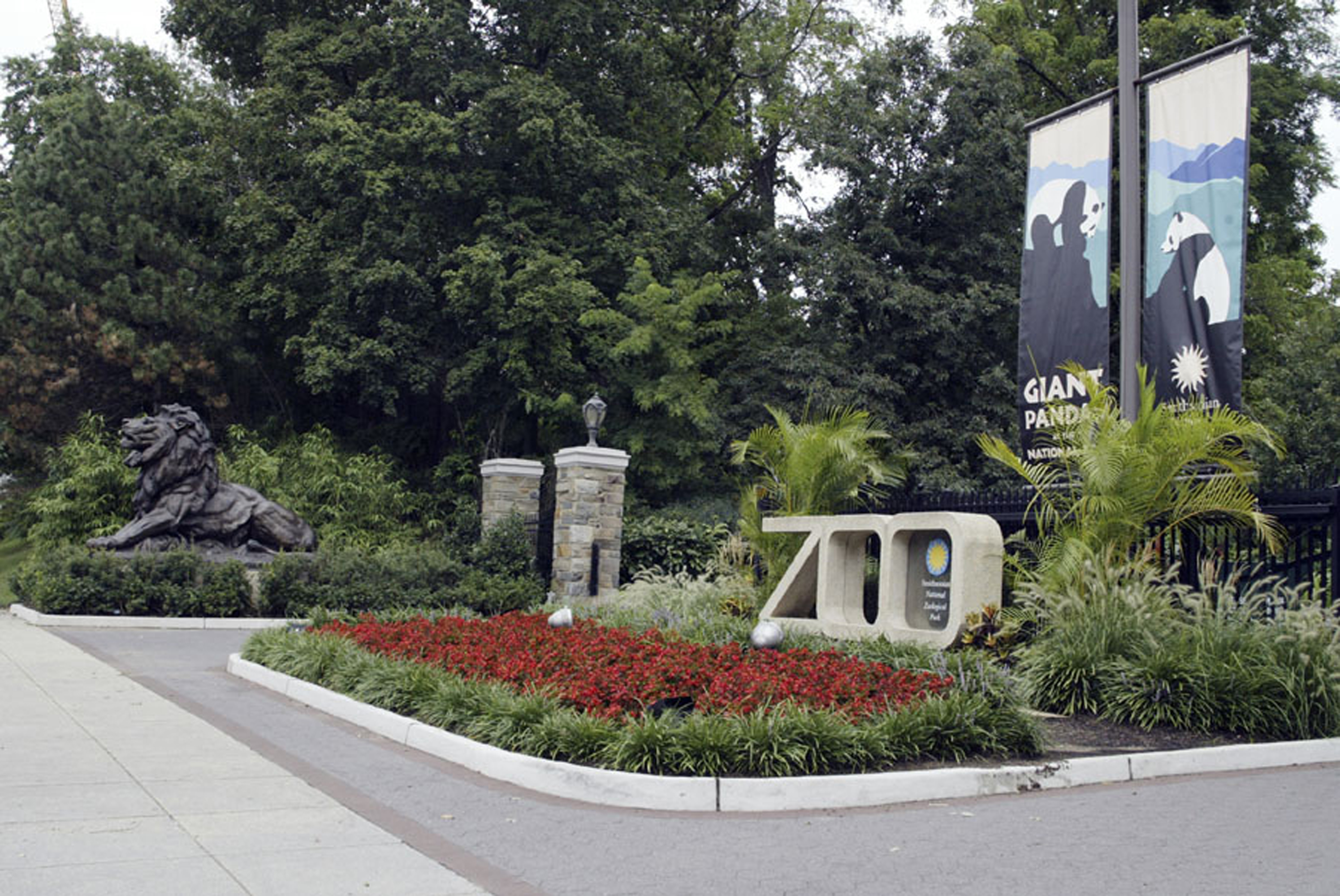This photograph captures what appears to be the entrance of a zoo, framed by a lush, landscaped area. Dominating the scene is a prominent stone sculpture that spells out "ZOO" in large, bold letters. Embedded within the second 'O' is a smaller informational placard, likely indicating the specific name or details of the zoo, though the text is not legible. Surrounding the sculpture, we see vibrant vegetation, including a notable patch of red flowers, adding color to the verdant setting.

To the left of the main sculpture stands an imposing black metallic statue of a lion, captured mid-roar, adding a dynamic focal point to the scene. On the right side of the photograph, a light pole adorned with colorful banners advertises a giant panda exhibit, featuring illustrations of two pandas perched on rocks.

The overall impression suggests a thoughtfully designed entryway intended to welcome and inform visitors, even though no people or animals are visible in the shot, emphasizing the serene yet inviting atmosphere of this zoo entrance.